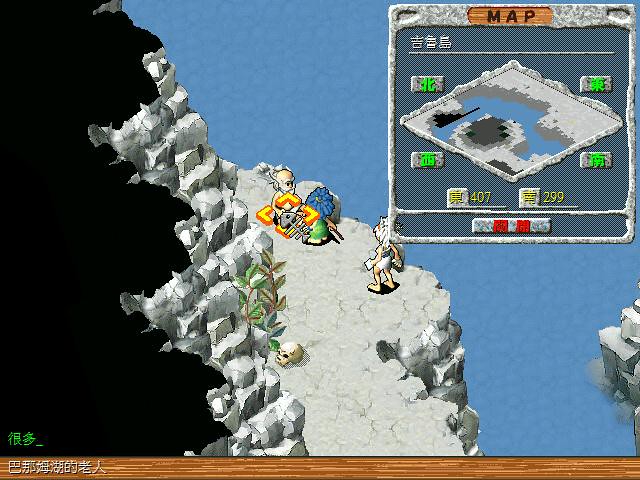The screen capture depicts a scene from a retro video game. At the center of the screen stands the main character, who is dressed in white shorts and gloves and is barefoot, adding to the unique detailing. The character's identity remains ambiguous, possibly human or an animal, contributing to the game's mysterious appeal. The game displays a clear influence of Asian culture, highlighted by the kanji-style text in white, positioned against a brown backdrop on the bottom left of the screen.

The graphics are indicative of an older game, with a somewhat primitive yet nostalgic appeal. The setting features a rugged, grey stone cliffside that runs parallel to a shimmering blue body of water. Additionally, a map located in the top right corner of the screen outlines various areas, confirming the character's current position by the water and suggesting proximity to a mountainous region.

In the foreground, there appears to be a vendor or a merchant, surrounded by fish bones and various items laid out in front. This element adds a lively touch to the environment, implying a marketplace or trading post within this cliffside locale.